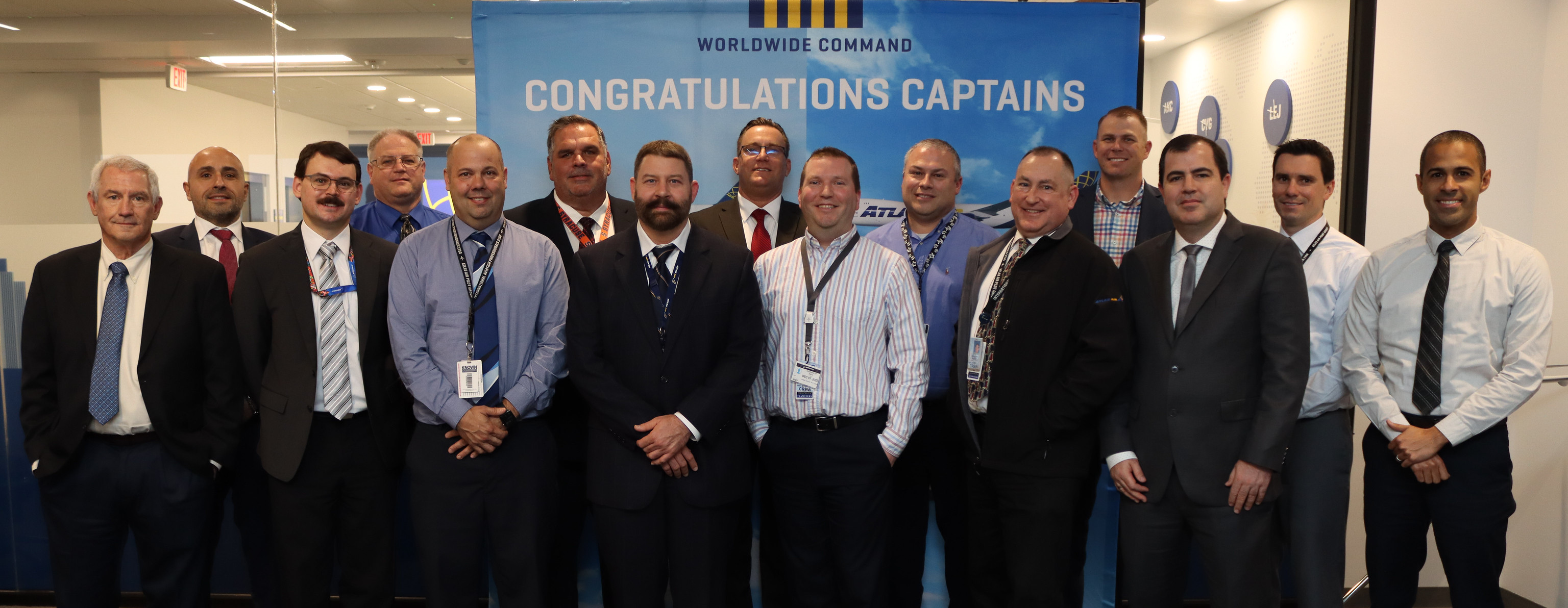The photo captures a group of approximately 15 to 20 men standing in two rows, posing for the camera. They are all dressed in formal office attire, with a mix of dark suits, white shirts, ties, and some sporting lanyards and badges. The backdrop features a large banner with a light blue sky and cloud motif. The banner prominently displays a vertical blue and yellow striped logo with the text "Worldwide Command." Below that, in large white block letters, it reads "Congratulations, Captains!" The scene is set in an office building, evident from the glass doors and hallway visible in the background. The composition suggests this could be a graduation or award ceremony for new airline captains.